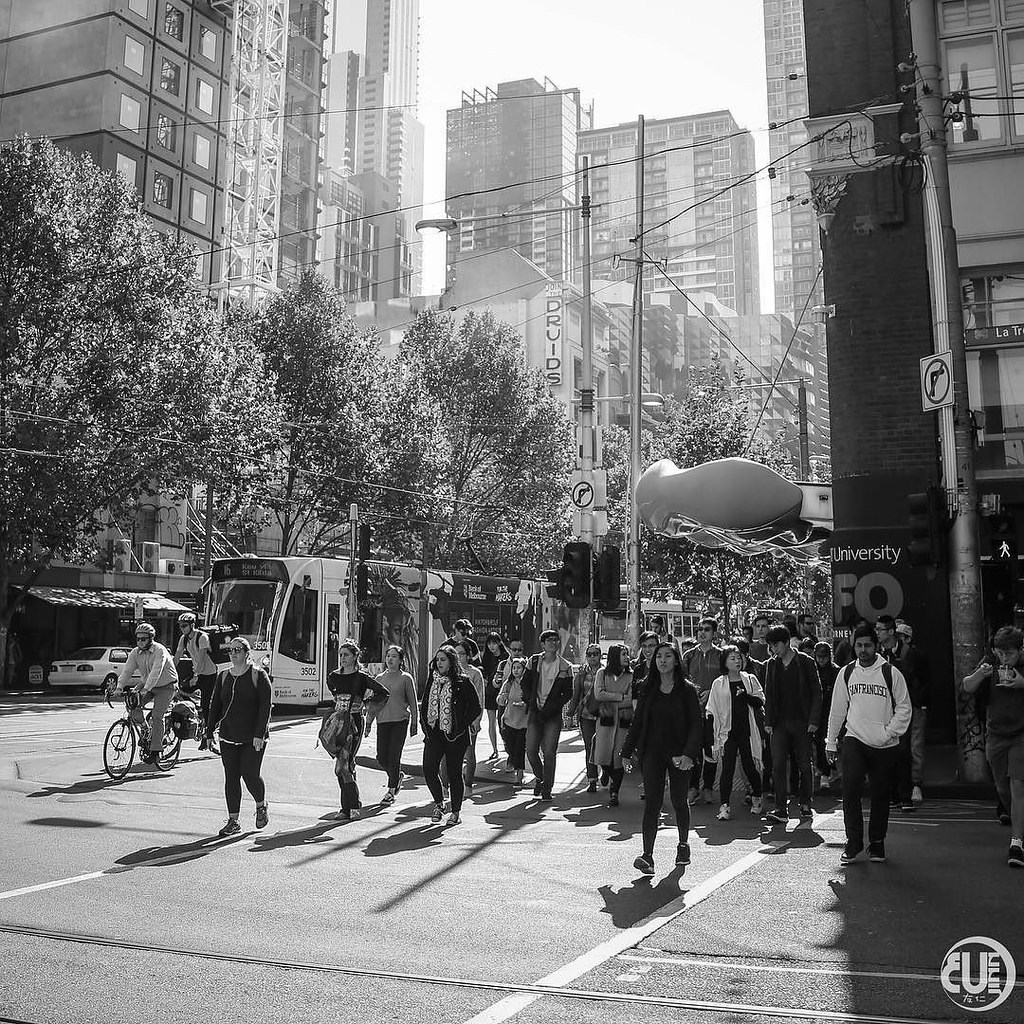This black-and-white photograph captures a bustling urban street scene with a diverse crowd of approximately 40 to 50 pedestrians crossing a wide intersection from the center-right to the lower-left. Among the crowd, a gentleman in a white hoodie with a backpack, and a woman at the forefront in a dark jacket stand out. Additionally, there are two cyclists navigating the crosswalk. In the midground, a trolley, connected to overhead wires, moves from right to left along its tracks, adding to the dynamic atmosphere.

The background features tall, possibly residential, buildings and a row of trees lining the street. The buildings have commercial establishments at ground level and offices above, with visible signage including the letters "DRVIDS" on one of them. Overhead, numerous wires are strung between telephone poles, one of which extends prominently up to the top of the photo. An area labeled "University" suggests an academic presence in the vicinity, while a "No Turn" sign adds to the urban detail. In the bottom right corner, a white circle with the letters "EU" is noticeable, possibly a part of some signage or street markings.